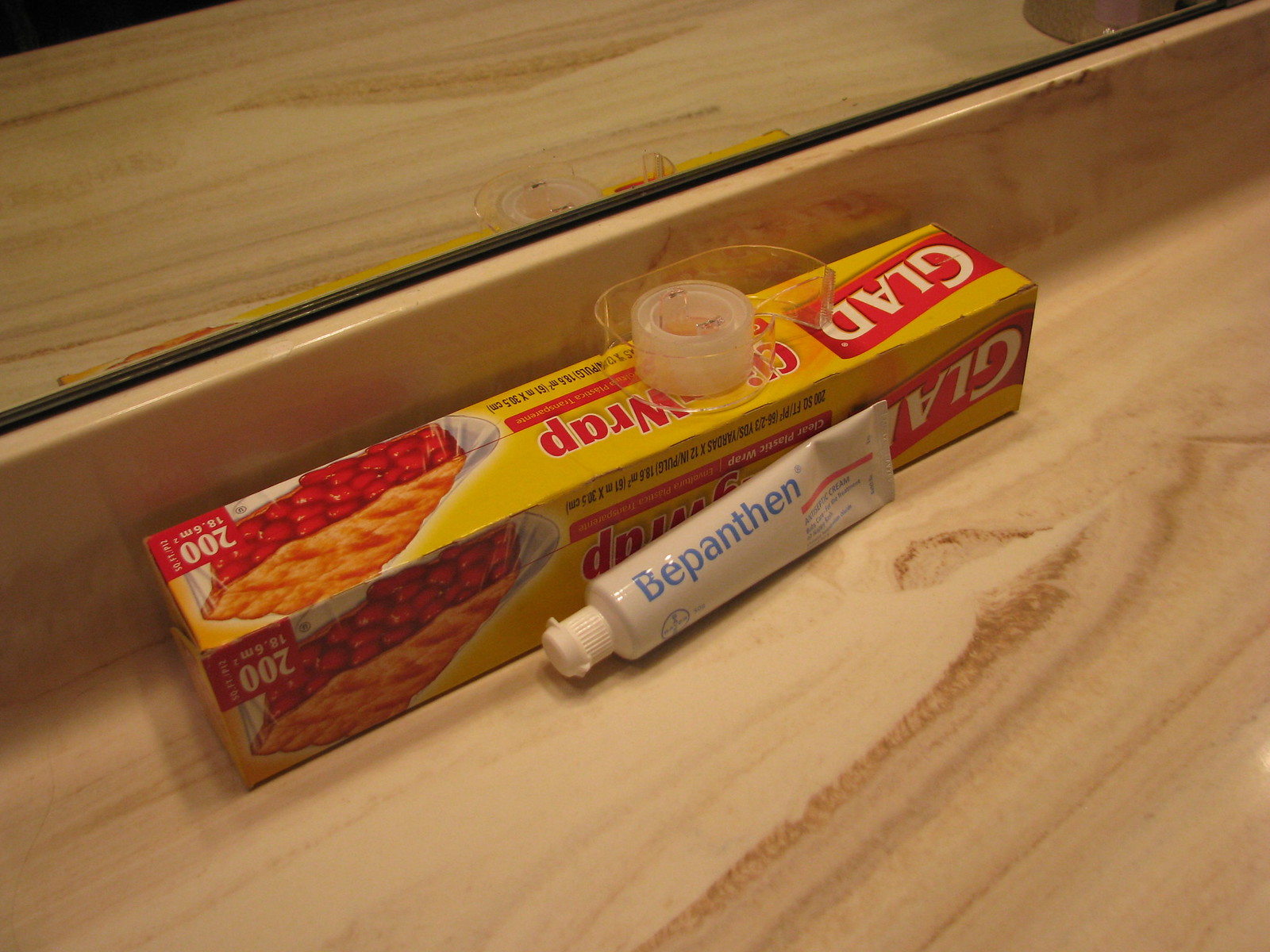A high-angle indoor color photograph captures a portion of what appears to be a bathroom countertop, inferred by the presence of a mirror starting diagonally from the center left edge and extending out of the frame in the upper right corner. The mirror's placement provides reflections that add depth and context to the scene.

The countertop, a tan marble with distinct grain patterns, is neatly arranged with several items against the backsplash. A rectangular box of GLAD cling wrap is prominently displayed, its label facing upside down to the viewer. On top of the box sits a clear cellophane tape dispenser, devoid of any labeling. In front of the box is a gray tube with a white cap, angled towards the lower left corner, bearing the blue-lettered inscription "Bepanthen," which hints at a topical cream.

The GLAD cling wrap box features bold white letters spelling out "GLAD" and "cling wrap" beneath it, with the upper left corner displaying "200" alongside an image of a wrapped piece of pie. The photograph is in sharp focus, although it suffers from poor lighting, resulting in subdued tones. The mirror contributes to the composition by reflecting the scene, enhancing the visual interest of the countertop arrangement.